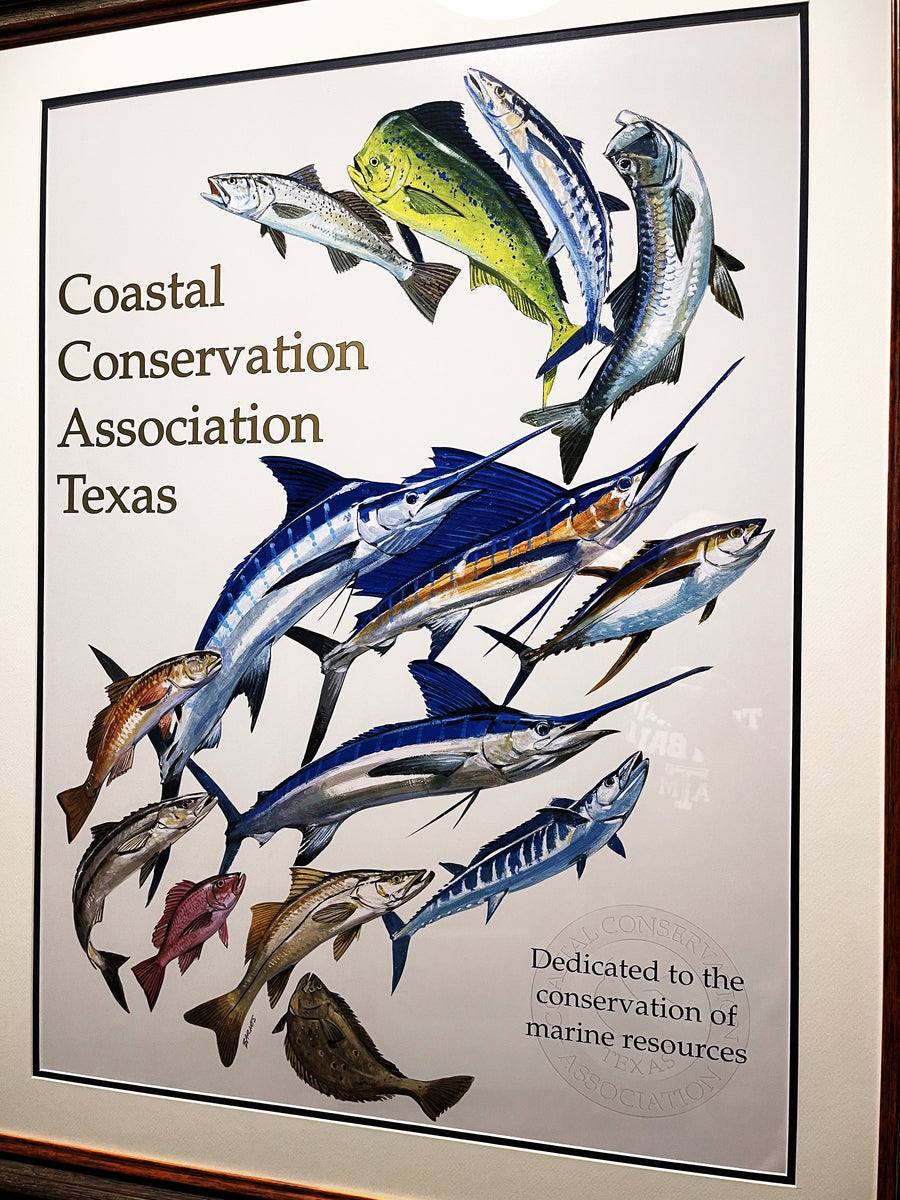Displayed within a brownish-red wooden frame, this captivating poster features a collection of vibrantly colored fish illustrations, reminiscent of watercolor art, set against a crisp white background. The inset border is black, adding a striking contrast to the composition. The large, bold text on the left-hand side reads "Coastal Conservation Association, Texas," with smaller dark blue text in the bottom right corner stating, "Dedicated to the Conservation of Marine Resources."

The fish, depicted in an array of colors including blue, pink, yellow, green, and brown, appear to swim in an elegant reverse S-shape across the poster. This fascinating lineup includes various species such as swordfish, marlin, grouper, tuna, barracuda, bass, ahi tuna, and skatefish. Notably, a pair of blue swordfish and a marlin with intricate browns and blues stand out amidst the plethora of aquatic life. Accompanying these aquatic illustrations, a circular seal in the bottom right further underscores the dedication to marine resource conservation in Texas.